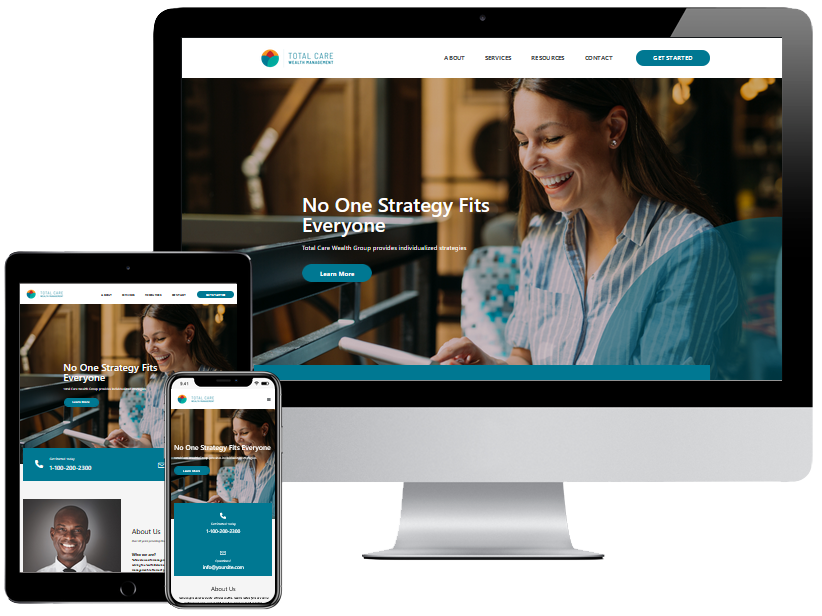The image showcases a gray or off-white computer monitor displaying the website "Total Care Health Management." The website interface includes navigation options such as About, Services, Resources, Contact, and Get Started, with the "Get Started" button highlighted in a greenish-blue color. Next to the "Total Care" title, there's a small circular icon featuring multiple colors: bluish green, blue, red, and yellow.

Prominently displayed on the screen is an image of a smiling Caucasian woman with long brown hair. She appears to be interacting with an iPad or cell phone, and she is dressed in a blue and white striped shirt. Beside her image, text reads, "No one strategy fits everyone. Your care, wealth, group providers, individualized strategies. Learn more." It looks like she is in the comfort of her home.

To the left of the computer monitor are a tablet and a cell phone, both displaying the same website. At the bottom of the phone screen, there is an African-American male smiling. The website provides a contact number, albeit difficult to read, likely 1-100-200-2300. The male figure's presence adds a personal touch, aiming to inform viewers about the company's services.